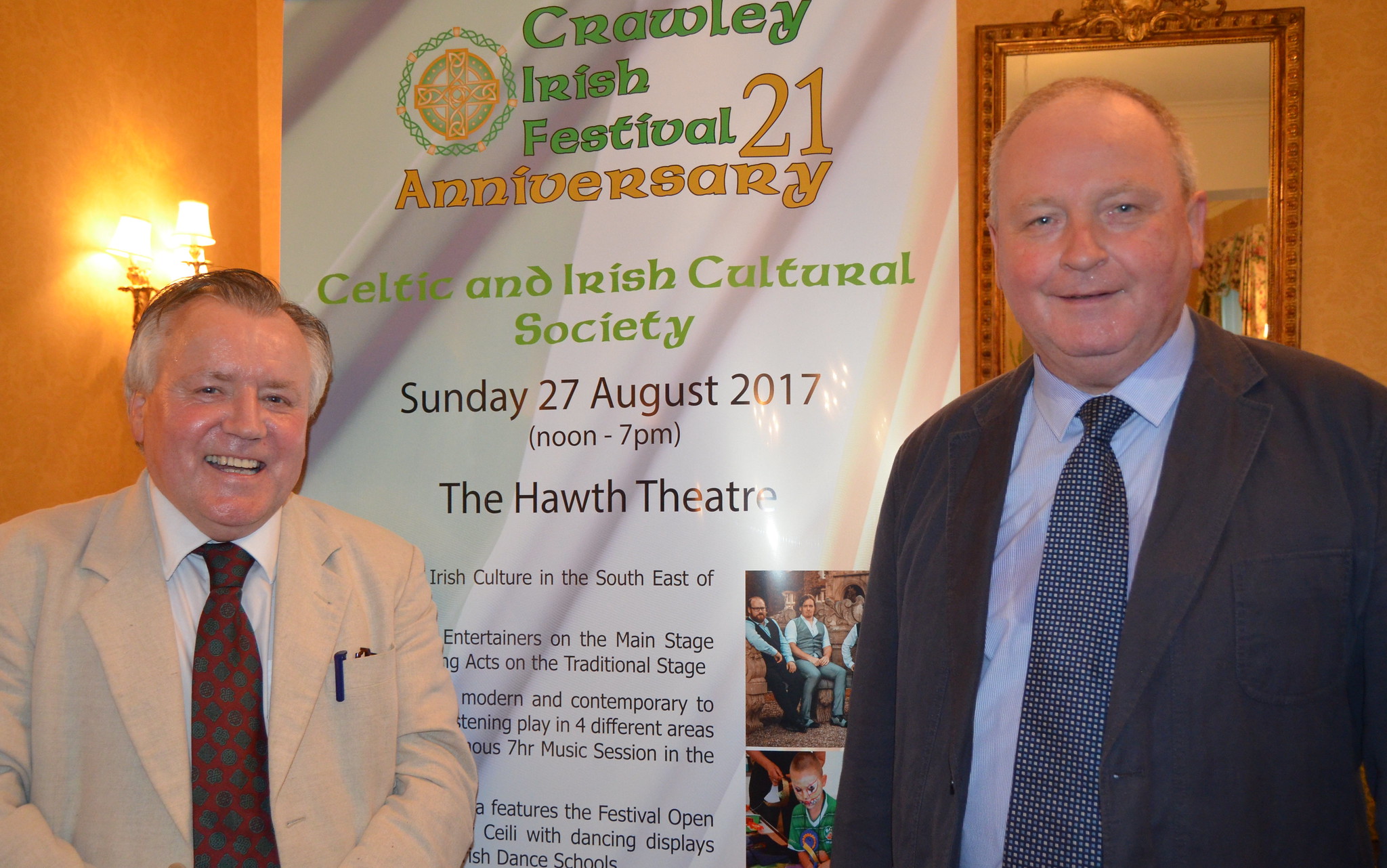The image features two older men standing in front of a yellowish-orange wall. The man on the left is shorter with brown and white hair, wearing a beige jacket, white shirt, and a reddish-brown tie adorned with green polka dots. He is smiling, and has brown-framed glasses with a blue pen in his pocket. The taller man on the right is balding and dressed in a blue suit jacket, blue shirt, and a blue tie. 

Between them hangs a white banner for the Crawley Irish Festival, featuring green and yellow lettering announcing the "21st anniversary" and the "Celtic and Irish Cultural Society." Additional text in black details the event date: "Sunday, 27 August 2017, noon to 7 pm at the Hoth Theatre," along with various festival activities, although some text is obscured. The banner includes small images, one depicting men in suits—one in a black suit with a blue shirt and another in a gray vest and blue jeans—along with a child in a green shirt.

The background shows yellowish walls with a mirror and a light fixture, alongside window views that reveal a blue sky. The setting is further detailed by a gold-trimmed picture frame and tan curtains. Additionally, a gold cross with green accents is visible on the banner, enhancing the Celtic theme of the festival.